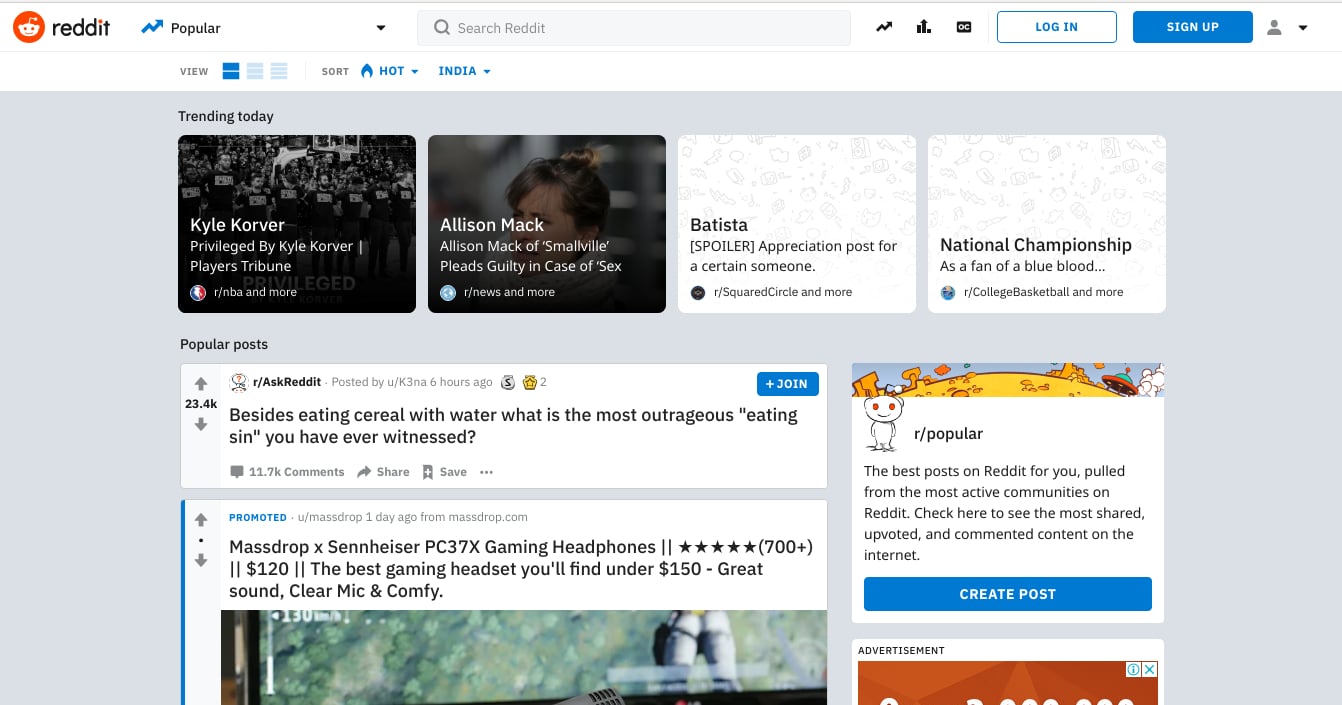This image captures a screenshot of the Reddit homepage. At the top of the page, the iconic Reddit logo is visible, featuring a small, smiling alien face within an orange circle, complete with an antenna. Next to the logo, the word "Popular" is displayed, accompanied by an upward-trending graph icon, signaling trending content. Beside the "Popular" section, there's a search icon available for users to find specific content.

Below the navigation bar, the "Trending Today" section highlights various trending articles. The first article's title is "Kyla Krova, privileged" authored by Kyla Krova on The Players' Tribune. The second article features a headline about Alison Mack from "Smallville," mentioning she has pleaded guilty in a significant case. Another article mentioned is titled "Batista Appreciation Post" with the word "spoiler" indicated in brackets. Additionally, there is an article about "National Champions" from the perspective of a "fan of blue blood."

On the main screen, the most popular post is prominently displayed at the bottom. This post poses a quirky question: "Besides eating cereal with water, what is the most outrageous eating sin you have witnessed?" Alongside this post, there is an advertisement for Massdrop x Sennheiser PC37X gaming headphones. The ad includes a five-star rating, the price of $120, and mentions that these are the best gaming headsets available under $150.